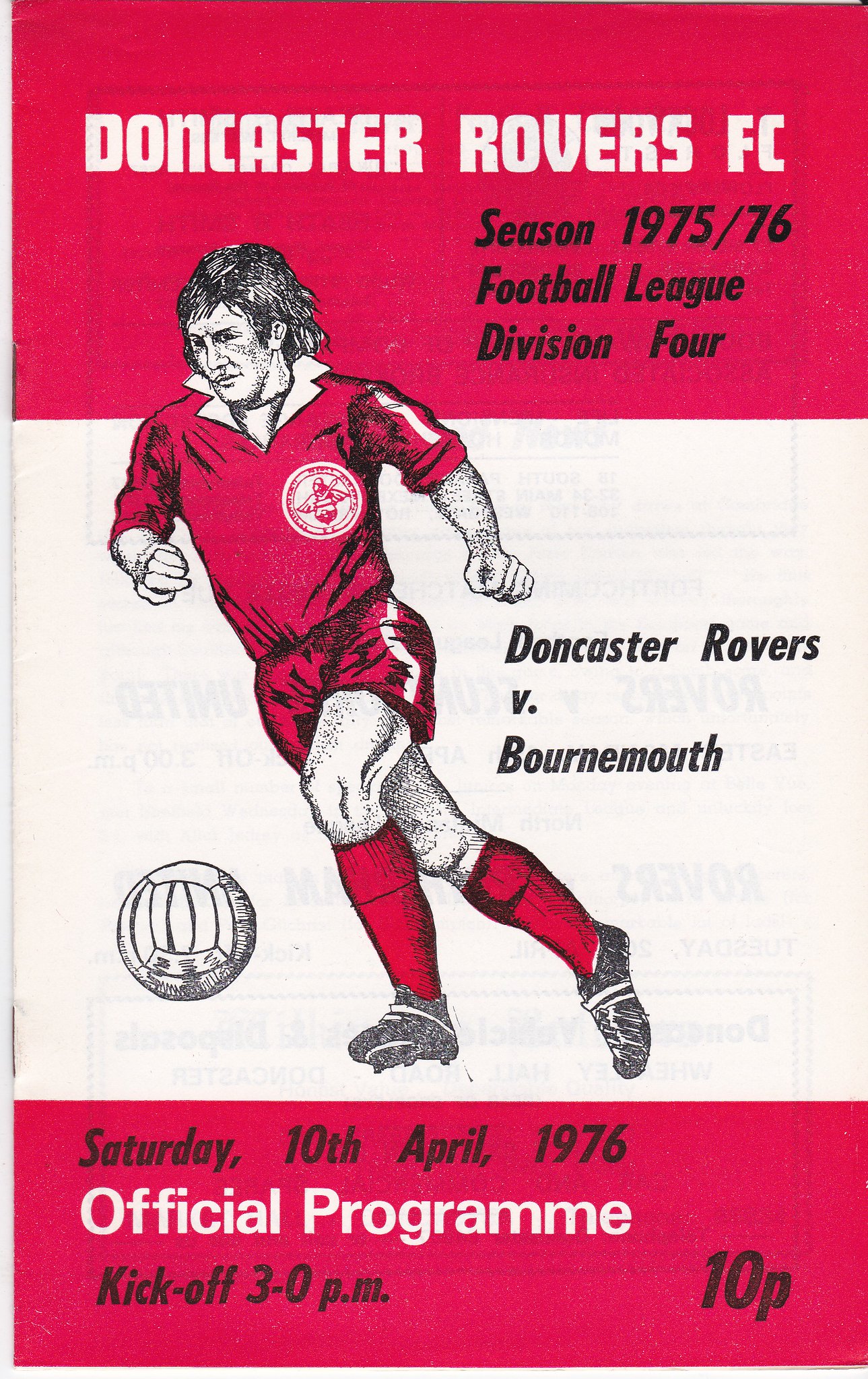The image is a program cover for a football match between Doncaster Rovers FC and Bournemouth, held on Saturday, 10th April 1976. The program is titled "Season 1975-76, Football League Division Four," which is printed in black letters. The design features a hand-drawn sketch of a man dressed in an all-red uniform, in the act of kicking a ball. Notably, the ball appears to resemble a volleyball more than a traditional soccer ball, with a distinct warped striping design instead of the classic honeycomb pattern. The cover is colored in red and white, and prominently displays the event details: "Official Program, kickoff 3 p.m." and the price "10 P" in the bottom right corner.